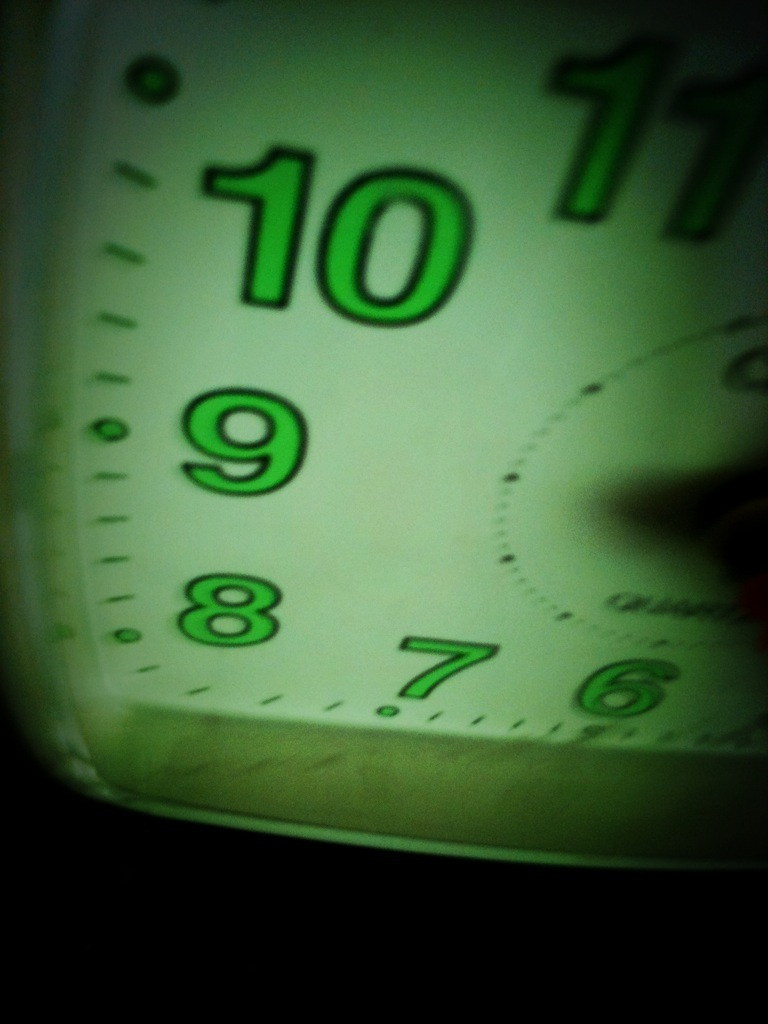The image depicts a close-up, angled view of a partially illuminated analog clock face in a dark room. The clock's numbers, ranging from 6 to 11, are prominently displayed in a neon green color with black outlines, suggesting they may glow in the dark. The face of the clock is white or has a whitish-green hue due to the green backlight. In the center of the visible part of the clock face, there is an inset displaying a smaller second clock with minute ticks and small circles marking the time, as well as some text, possibly the brand name. A light shines on the main clock body, which appears to be made of metal, showing fine scratches, while the upper right and lower parts of the image remain in shadow, emphasizing the clock's luminescence. There are no visible minute, hour, or second hands in this photograph, enhancing the focus on the clock's illuminated numbers and intricate details.